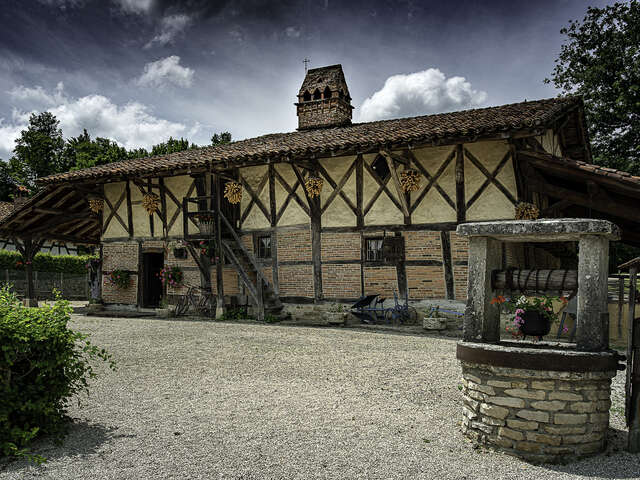This stylized photograph captures an old, multi-room cottage bathed in a surreal, almost dark blue sky with patches of puffy white clouds. The house, a two-story building, has a brick bottom and is topped with timbered beams. The house's cream and brown tones are accentuated by its unique architectural features, such as the small tower in the center with three openings and hanging baskets draped from the second-floor roof. Framed by green trees and a bush on the bottom left, the foreground features a historic brick-and-concrete wishing well, adorned with a floral hanging basket. The setting is grounded on a surface that appears to be made of small pebbly stones, adding to the rustic charm of the scene.